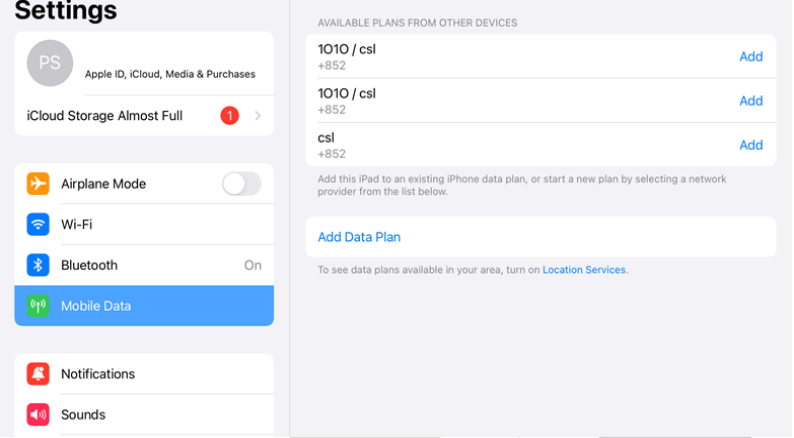The screenshot displays a detailed view of the settings menu on an iPhone. On the left side, the menu options are arranged vertically, starting with "Settings" at the top. Below that, there's a circular icon labeled "PS," followed by "Apple ID, iCloud, Media & Purchases." The next item is a warning in red text, "iCloud Storage Almost Full." Continuing down the list are other settings: "Airplane Mode," "Wi-Fi," "Bluetooth," and "Mobile Data," the latter highlighted in blue to indicate its current selection. The subsequent options are "Notifications" and "Sounds," each accompanied by corresponding icons on their left.

On the right side of the screen, a larger rectangular section is displayed with the title "Available Plans from Other Devices" at the top. The first listing is "1010/CSL +852," with the "Add" button positioned on the right. This is followed by a second listing, identically labeled "1010/CSL +852," also featuring the "Add" button on the right. The final option reads "CSL +852," again with the "Add" button adjacent to it.

Beneath these options, in smaller text, is a prompt: "Add this iPad to an existing iPhone data plan or start a new plan by selecting a network provider from the list below." Below this prompt lies an "Add Data Plan" button, accompanied by another snippet of small text that reads: "To see data plans available in your area, turn on location services."